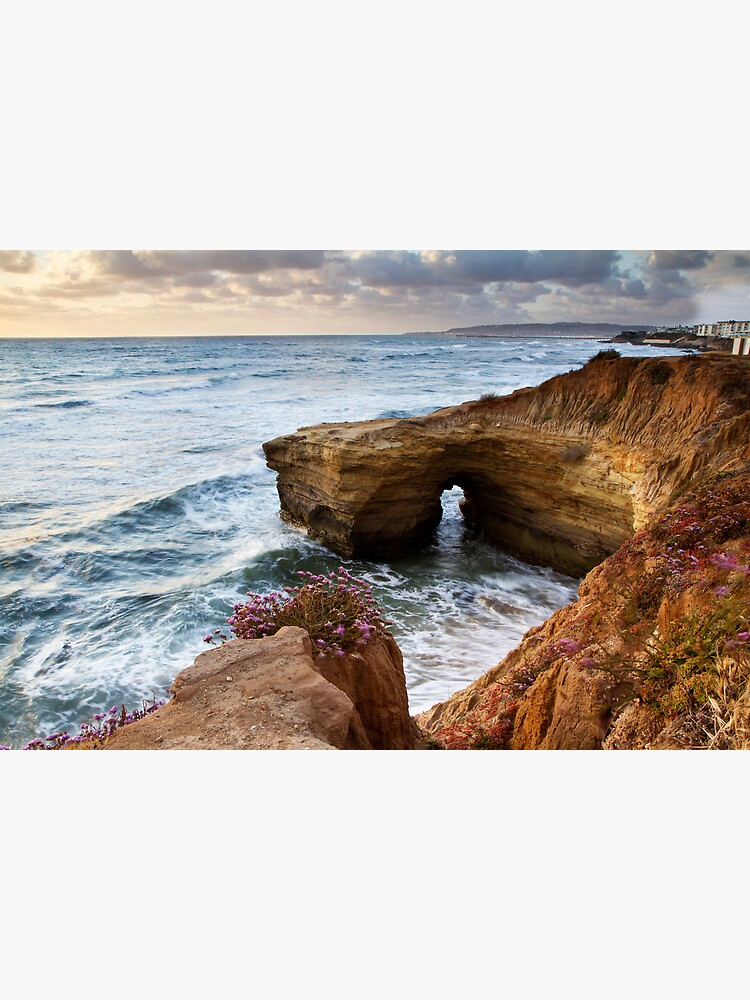This photograph captures a dramatic coastal scene during the day, with the sun low in the sky, illuminating the landscape in warm, yellowish light while dark gray storm clouds loom above. The main focus is a rugged, rocky cliff face composed of dark to light brown sandstone, stretching off the edge of the shore. Arched and jagged from eons of erosion, a distinct natural archway carved by the turbulent sea stands towards the center-right of the image, inviting the viewer to imagine walking through it. Crashing waves and frothy white water reveal the ocean’s turmoil, a dark greenish expanse of turbulent waves that fades into the distance under the brooding sky.

At the cliff's base and scattered throughout the rocky terrain are clusters of hardy, scrubby bushes adorned with vivid purple flowers, adding a splash of color against the earth tones. These resilient plants cling to the jagged cracks and crevices of the cliffs, accompanied by a few reddish vegetation spots. In the far background on the right, the silhouette of a distant coastline comes into view, dotted with what look like small, whitish buildings, their detailed features obscured by the distance and atmospheric haze. This image captures the raw, untamed beauty of nature juxtaposed with the faint whisper of human presence far off in the horizon.